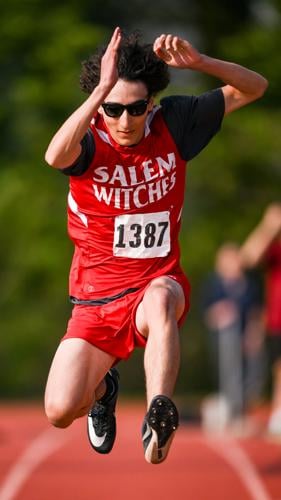In the image, a track and field athlete is captured mid-air against a blurred, greenish background of trees. The reddish track with white lines is visible beneath him. A few spectators are standing to the right, watching him. The athlete, with flowing long black hair and tinted black sunglasses, is airborne with both feet off the ground. His hands are raised near his forehead, palms up. He is donned in a black t-shirt beneath a red and black jersey emblazoned with "Salem Witches" in white. The jersey also has a white rectangular number tag with "1387" in black. He wears short red athletic shorts and black and white running shoes. The photo, with its tall and focused composition, captures the dynamic motion of his jump, emphasizing the athletic prowess and intensity of the moment.